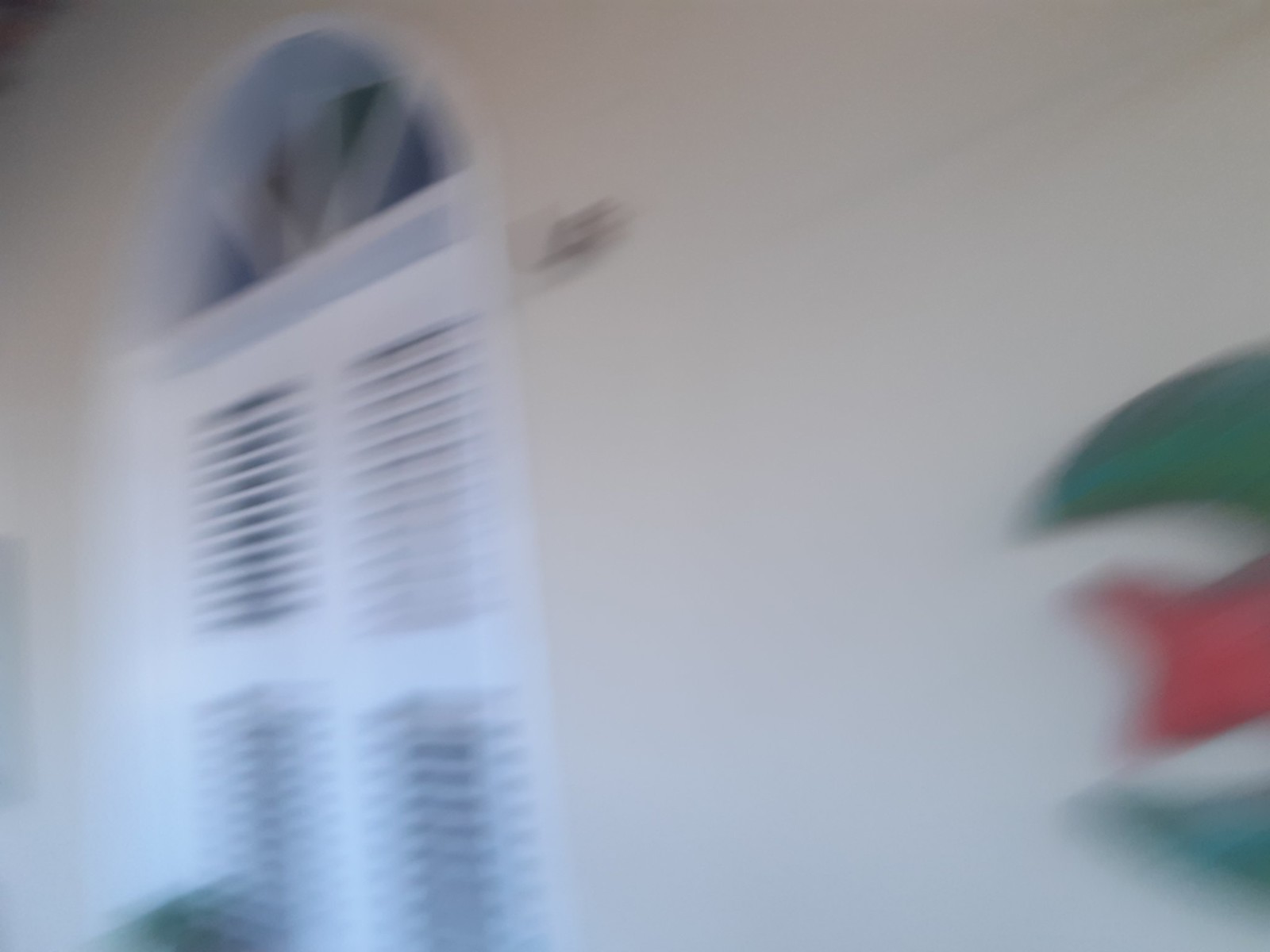This photograph captures a blurred view of what appears to be the front or side of Simone's home, showcasing its distinctive architectural style. Prominently featured are closed white shutter windows with a charming curved arch at the top, designed in a way that suggests adjustable blinds to allow airflow. The exterior wall, painted in a soft cream color, provides a serene backdrop. Within the frame, there’s also a green, curved symbol resembling either a fish or a claw with a red central element, possibly a tongue, though these details are blurred. The combination of these elements evokes a cozy, artistic ambiance typical of this residence.